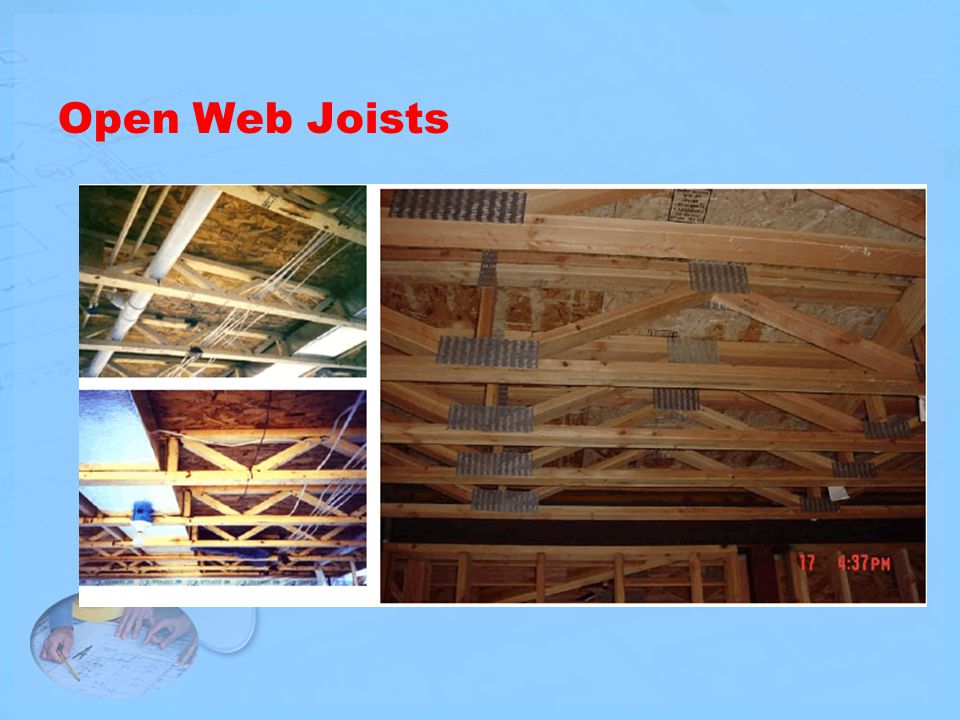The image is a PowerPoint presentation slide depicting "Open Web Joists" as indicated by the red text at the top on a light blue background. The slide is composed of three photographs showcasing ceiling joists in a construction setting. On the left, there are two smaller images stacked vertically, capturing close-up views of ceiling areas with joists. The right side features a larger image that provides a broader perspective of the ceiling structure. The joists appear to consist of large wooden beams, where two horizontal beams are placed parallel, one directly under the roof and another at a distance below. These beams are connected by smaller diagonal wooden beams creating an alternating pattern that securely supports the ceiling. Additionally, the presentation slide includes a timestamp at the bottom left corner reading "17:37 PM," and a small circular inset image of hands holding a pencil and working on a keyboard, located below the main images. The colors throughout the slide include light blue, red, brown, light brown, tan, and yellow, giving the overall layout a detailed and professional presentation aesthetic.